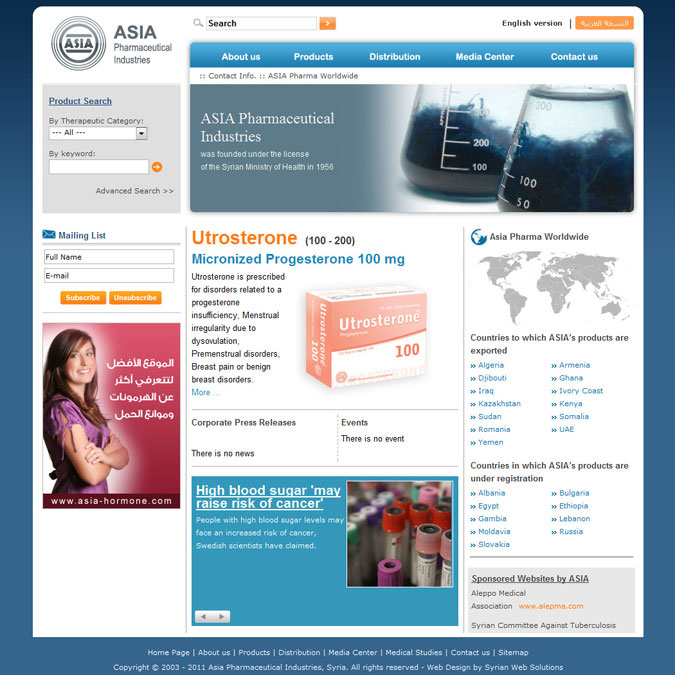The image is a screenshot likely taken from a website, possibly viewed on a tablet or laptop, given its square shape. The entire background of the screenshot is blue. Along the bottom, from the bottom left to the bottom right, there is a footer containing links labeled: "Homepage," "About Us," "Products," "Distribution," "Media Center," "Medical Studies," "Contact Us," and "Sitemap." Below these links, the footer also reads, "Copyright, 2003 to 2011, Asia Pharmaceutical Industries, Syria. All rights reserved," with credit for the web design given to "Syrian Web Solutions."

The rest of the webpage is dominated by a white block. In the upper left-hand corner, it displays the name "Asia Pharmaceutical Industries," accompanied by the company's logo. A search bar is positioned near the top, along with an indication in the upper right corner that the content is in the English version, with an orange button offering the option for an Arabic version.

Below the navigation bar, there's a row of light blue tabs labeled: "About Us," "Products," "Distribution," "Media Center," and "Contact Us." Directly beneath these tabs, the text "Contact Invo, Asia Pharma, Pharma, Worldwide" is displayed. The main content area features a prominent image accompanied by text on the left side that reads: "Asia Pharmaceutical Industries was founded under the license of the Syrian Ministry of Health in 1956." To the right, there are two science lab bottles with dark blue, active, fluffy ingredients swirling inside them.

Below this section, there are multiple columns containing various pharmaceutical products, including "Eutrosterone" and "Micronized Pregnazone," each with accompanying images. The entire page is dedicated to pharmaceutical information and products.